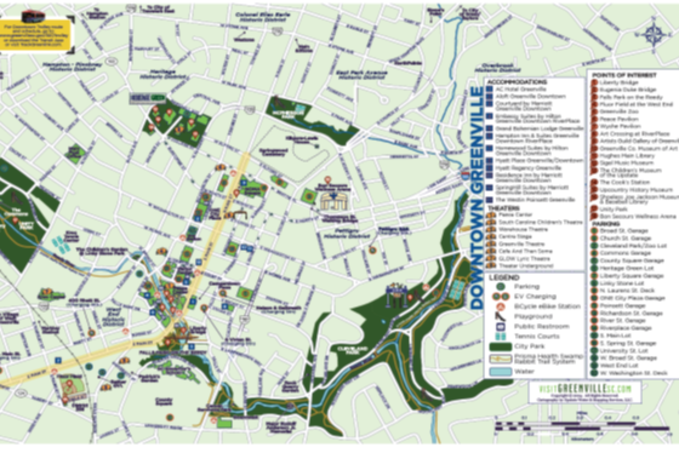The image is a low-resolution scan of a city map, likely a visitor guide or brochure for downtown Greenville. The map predominantly features pale green buildings of various shapes with white lines representing streets in a grid-like pattern. A prominent yellow line, possibly indicating a train or bus route, extends from the lower left corner through the center and towards the top of the image. On the right-hand side, there is a blurry map legend that includes rows of blue squares with text, followed by orange symbols with accompanying text. The legend's text starts with the word "Legend" itself, but the rest is too blurred to read. Vertically aligned on the left side, bold blue block letters spell out "Downtown Greenville." The map also includes several green areas, a scale for distances in the bottom right corner, and a compass indicating cardinal directions in the top right. In the top left-hand corner, there is an unreadable yellow box with black text.